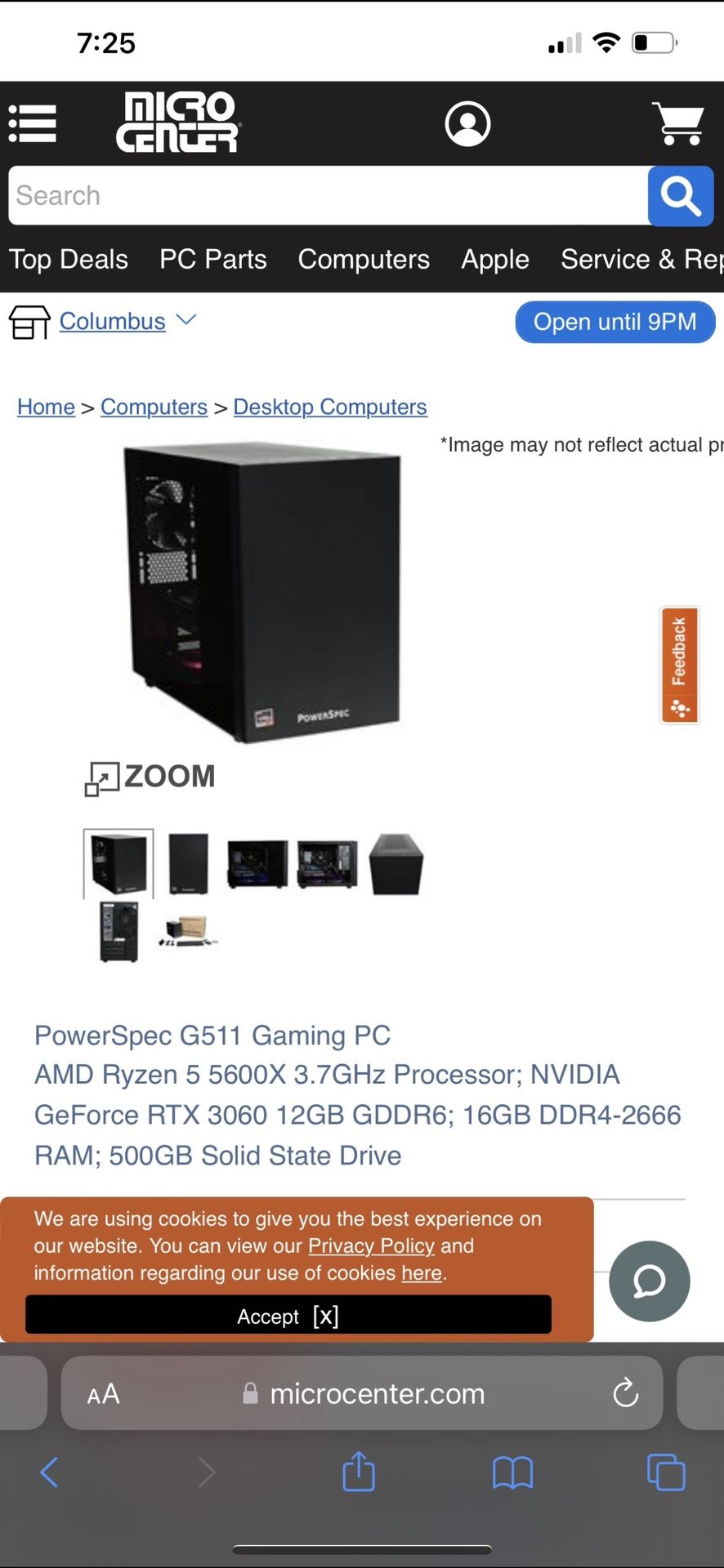The image is a screenshot from a website dedicated to computer parts and systems, presumably from Micro Center. At the top of the page, the time reads 7:25, accompanied by icons indicating battery status, internet connectivity, and phone signal. The Micro Center logo is prominently displayed, with options to access the user profile and shopping cart nearby.

Just below the header, there's a search bar for user queries. Navigation tabs include links to top deals, PC parts, computers, Apple products, services, and repairs. A dropdown menu indicates the selected store location as Columbus. Adjacent to this is a blue, pill-shaped box displaying the store hours: "Open until 9PM."

The breadcrumb trail provides navigation context, listing "Home > Computers > Desktop." The main section of the screenshot features a product image and a disclaimer about the accuracy of the image. The featured product is a PowerSpec G511 gaming PC, which is shown being black and square with a visible fan. Users are given the option to zoom into the image, and there are seven smaller thumbnail images displaying the product from various angles.

Below the product images, the detailed listing reads: "PowerSpec G511 Gaming PC - AMD Ryzen 5 5600X 3.7GHz Processor." The footer of the page includes a cookie usage notice with links to view the privacy policy and cookie information, along with options to accept or decline the use of cookies. There is also an interactive element allowing users to leave a comment or engage with customer service.

Finally, the website URL, "microcenter.com," is displayed at the bottom of the page.